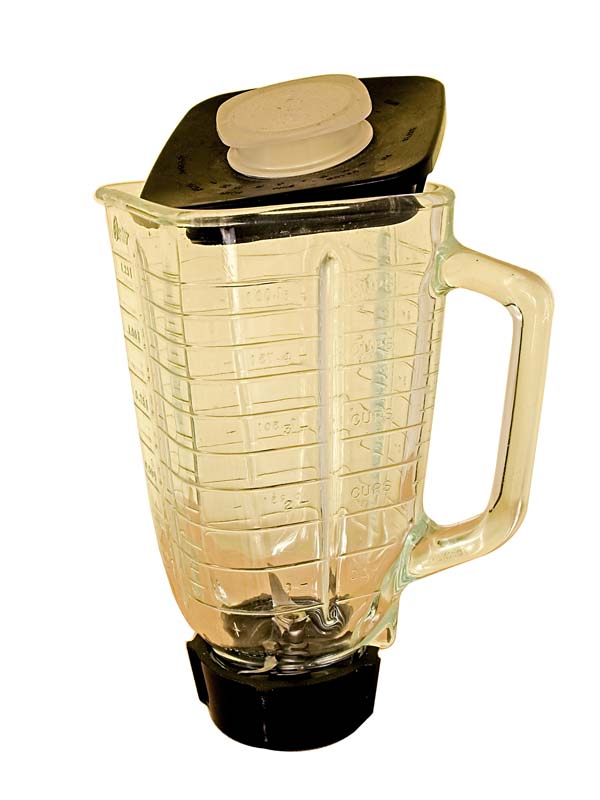This image features a blender jar cropped out of its natural context, with no motor or base visible. The clear glass container, which has a beige or tan tint, is detailed with measurement markings and the word "CUPS" visible on its surface. The jar features a prominent handle on the right side, running almost the entire height of the container. The jar is capped with a black lid that has a dark yellow circular notch for easy removal, though it's slightly askew. Inside the container, silver-toned blades affixed to a small circular black base are visible. The overall image appears to have a sepia-like tone, enhancing the vintage aesthetic against a plain white background.